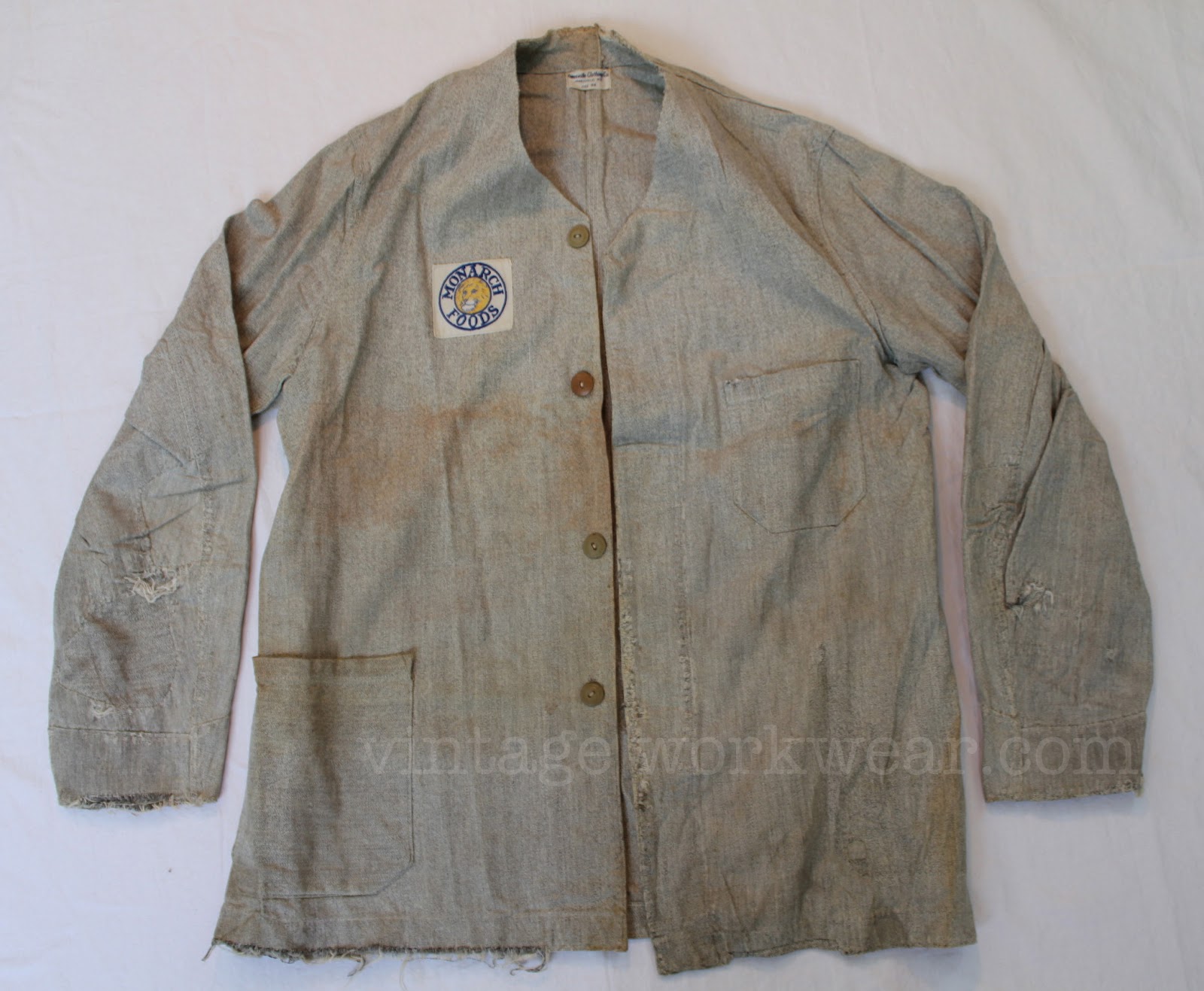This image captures an extremely well-worn vintage shirt, possibly a uniform or lab coat, associated with Monarch Foods. The shirt is a grayish-blue button-up, long-sleeved and bears significant wear and tear, with numerous stains and frayed stitching along the edges. It features patches sewn into the sleeves, indicative of attempts to mend and prolong its usability. There is a distinct white label with blue writing on the left breast pocket area, depicting the text "Monarch Foods" arched above and below a round yellow figure, resembling a sun or moon with a face on it. On the right side of the chest, there's another emblem with a smaller emblem below it. This shirt also has a larger hip pocket, and underneath that, lightly lettered, the text vintageworkwear.com can be seen. The blue background of the photo contrasts with the shirt, highlighting its tattered state and the holes in various places, particularly on the sleeves. This garment clearly saw extensive use and has an aura of historical labor.